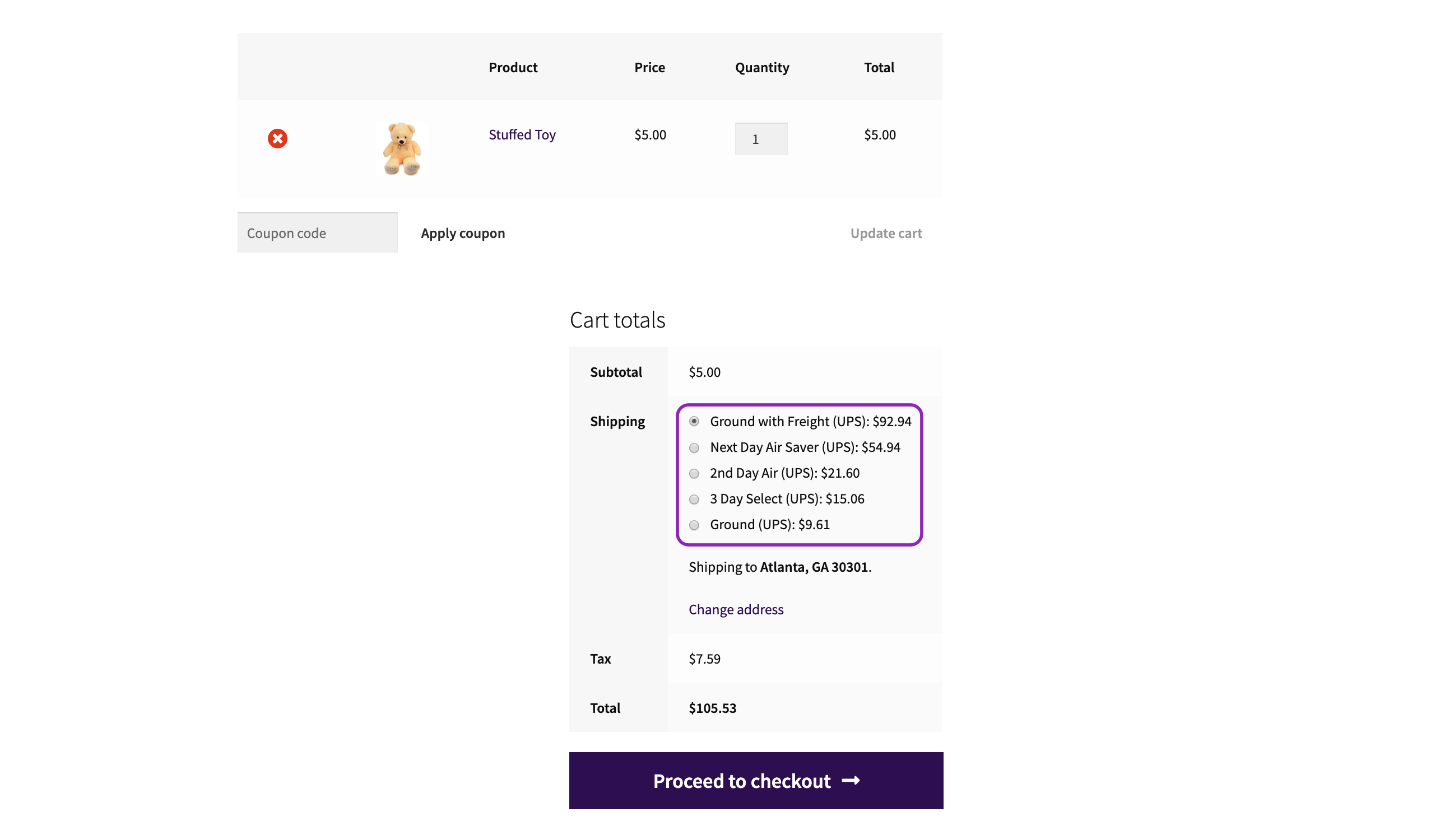Screenshot of an E-Commerce Checkout Page for a Stuffed Toy:

The image captured is a screenshot of a checkout page from an unnamed e-commerce website. At the top of the page, there is a very light grey bar that delineates the sections for "Product," "Price," "Quantity," and "Total."

Below this header is a lighter grey section featuring a red circle with a white "X" in the center, typically used to remove items from the cart. Adjacent to this icon is a thumbnail image of a tan stuffed bear, labeled "Stuffed Toy." The product name is in purple text, indicating that the link has been visited.

Underneath the "Price" column, the cost of the stuffed toy is listed as $5. The "Quantity" field displays a value of 1, and consequently, the "Total" is calculated as $5.

Just below the product image and details, there is a section for applying a coupon code, accompanied by a button to apply the discount. To the right of this coupon code section, another button labeled "Update Cart" is located beneath the total price of $5.

Further down, the "Cart Totals" section begins with a subtotal of $5. The shipping options are extensive, providing several options with their respective costs:
- Ground Freight UPS: $92.94 (selected by default)
- Next Day Air Saver UPS: $54.94
- Second Day Air UPS: $21.60
- Three Day Select UPS: $15.06
- Ground UPS: $9.61

Shipping is configured to Atlanta, Georgia, with the ZIP code 30301. There is a clickable link in purple text allowing users to change the shipping address if needed.

Following the shipping options, tax is calculated to be $7.59. Adding all these charges, the grand total sums up to $105.53. At the bottom of the page, there is a prominent purple button with white text that says "Proceed to Checkout."